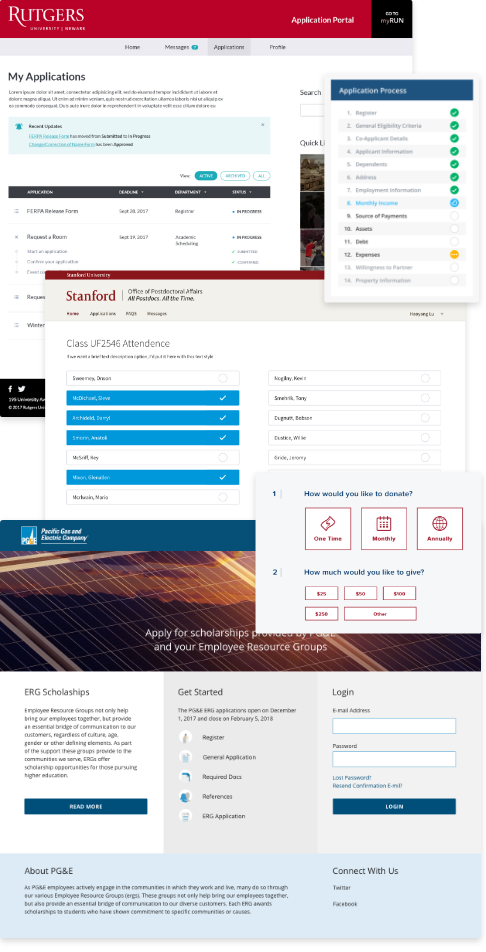The image showcases a cluttered visual collage of various application-related web pages. Dominating the top of the image, a red banner reads "Rutgers Application Portal," indicating the section of a busy university website. Below, a navigation menu featuring tabs like "Home," "Messages," "Applications," and "Profile" is visible, with the focus on the "Applications" section. This section is titled "My Applications", detailing the user's progress through the application steps. A progress tracker on the right reveals that the user is on step 8 out of 14, suggesting they are more than halfway through the application process. 

Adjacent to the Rutgers portal is a separate web page from Stanford, depicting a visual related to class attendance. Additionally, fragments of the Pacific Gas and Electric Company website are noticeable, specifically featuring an "Apply for Scholarships" section. The amalgamation of these disparate pages into a single image suggests a theme centered around various forms of applications. The collage-style assembly indicates a busy, multifaceted process, showcasing the user’s engagement with multiple important tasks simultaneously.